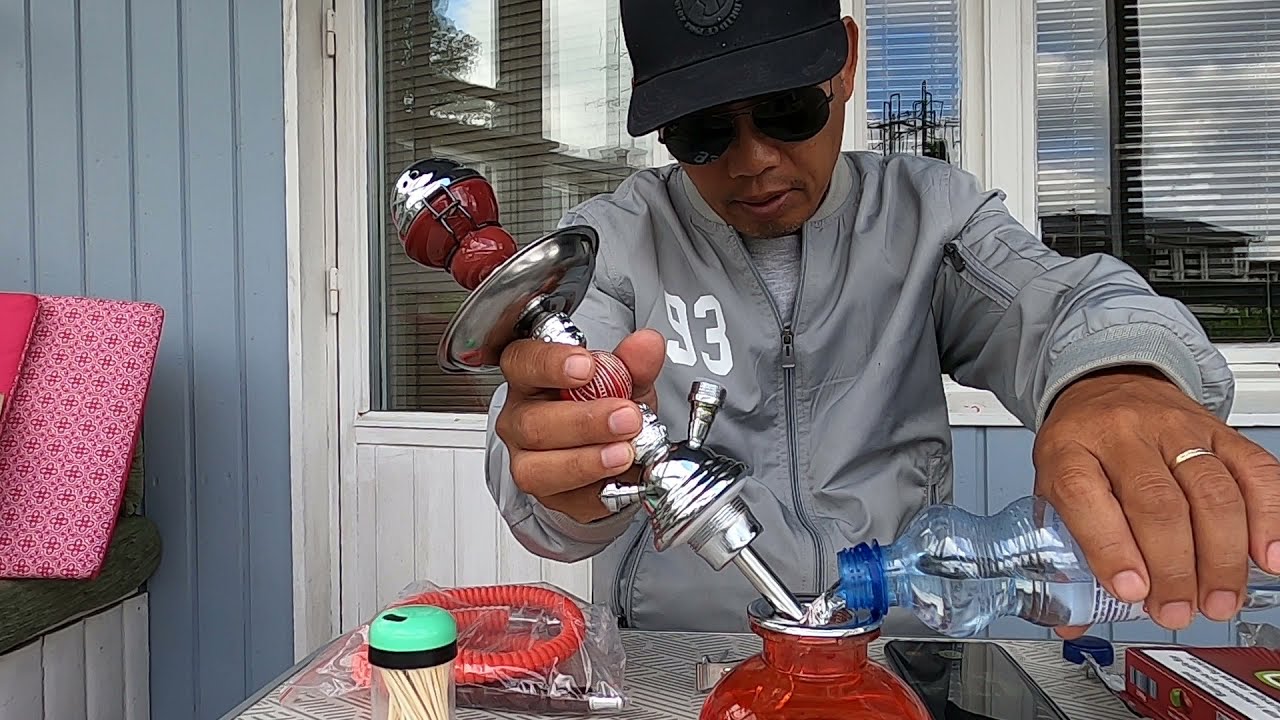A man, identifiable by his black cap and dark sunglasses, is seated at a table with various items. He wears a silver-gray jacket emblazoned with the number 93 in white. With a ring on his left finger, he holds a bottle of water, pouring it into an orange drink mixer that features a dark red cap. The table in front of him displays a range of objects: a black cell phone near the right edge, a small container of q-tips, toothpicks, and a red tube in a ziplock bag. Behind him, the setting includes light-patterned tables and a window with white frames and blinds. The exterior of the building is painted blue and white, complemented by grayish-blue siding. Adjacent to the man is a seating area with gray and pink cushions, enhancing the vivid and detailed ambiance of the scene.